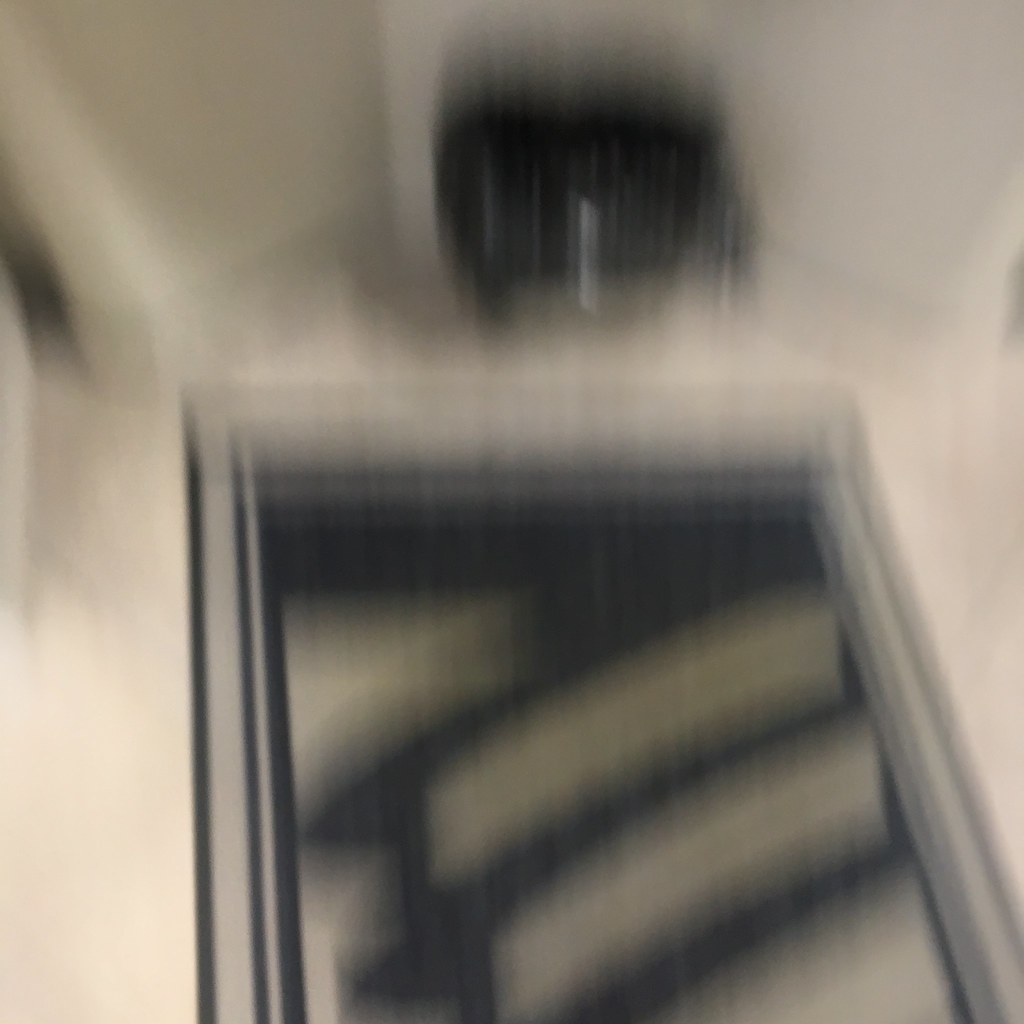This is a photograph marked by significant blurriness and a perplexing scene. At the center of the image, there appears to be a rectangular black object with white features, bordered in black, resembling a picture frame or a photograph laid flat on a surface. Surrounding this object is the floor or carpet, which is predominantly white, causing the object's edges to blend somewhat with the background due to the blur.

On what seems to be the upper portion of the photograph, there's an indistinct black item. Around this item is what appears to be a frilly cloth or curtain, adding to the mystique of the scene. To the left side, either a doorway or a mirror reflection comes into view. This framing object has a kind of grey outline, with the ceiling above it appearing mostly white. In what could be the reflection, or through the doorway, are curtains gathered against a wall, though this detail is equally obscured by the photograph's lack of focus. 

The overall composition of the image, from the intersecting lines of the rug on the floor to the complex interplay of light and objects above, creates a disorienting but intriguing visual narrative.